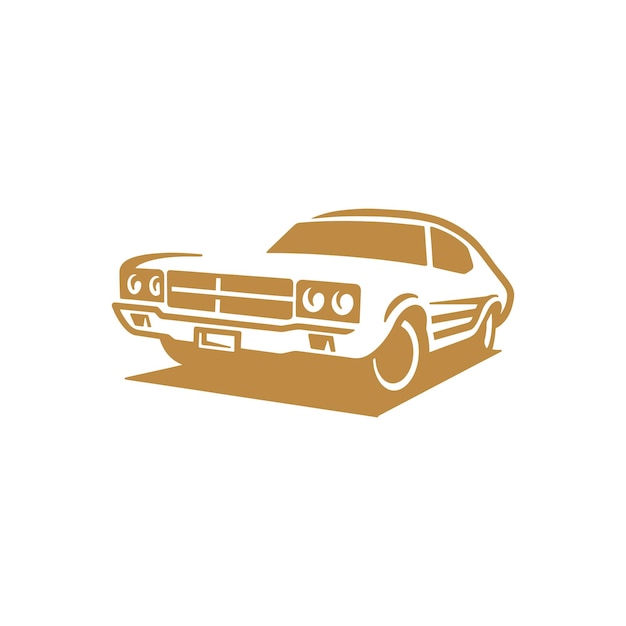The image features a minimalist drawing of a sporty car, likely a Ford Mustang hatchback or fastback. The car is depicted using light brown and white colors, with its outline and details sketched in a simplistic style. It has a prominent front grille, four headlights (two on each side), and black wheels, emphasizing the car's sporty appearance. The car, shown in a slanted position facing the bottom left, has two doors and windows outlined in brown. Below the car, there is a rectangular brown shadow against a white background. The entire composition is devoid of any text or intricate detailing, giving it a clean and straightforward look akin to a decal or a sticker.